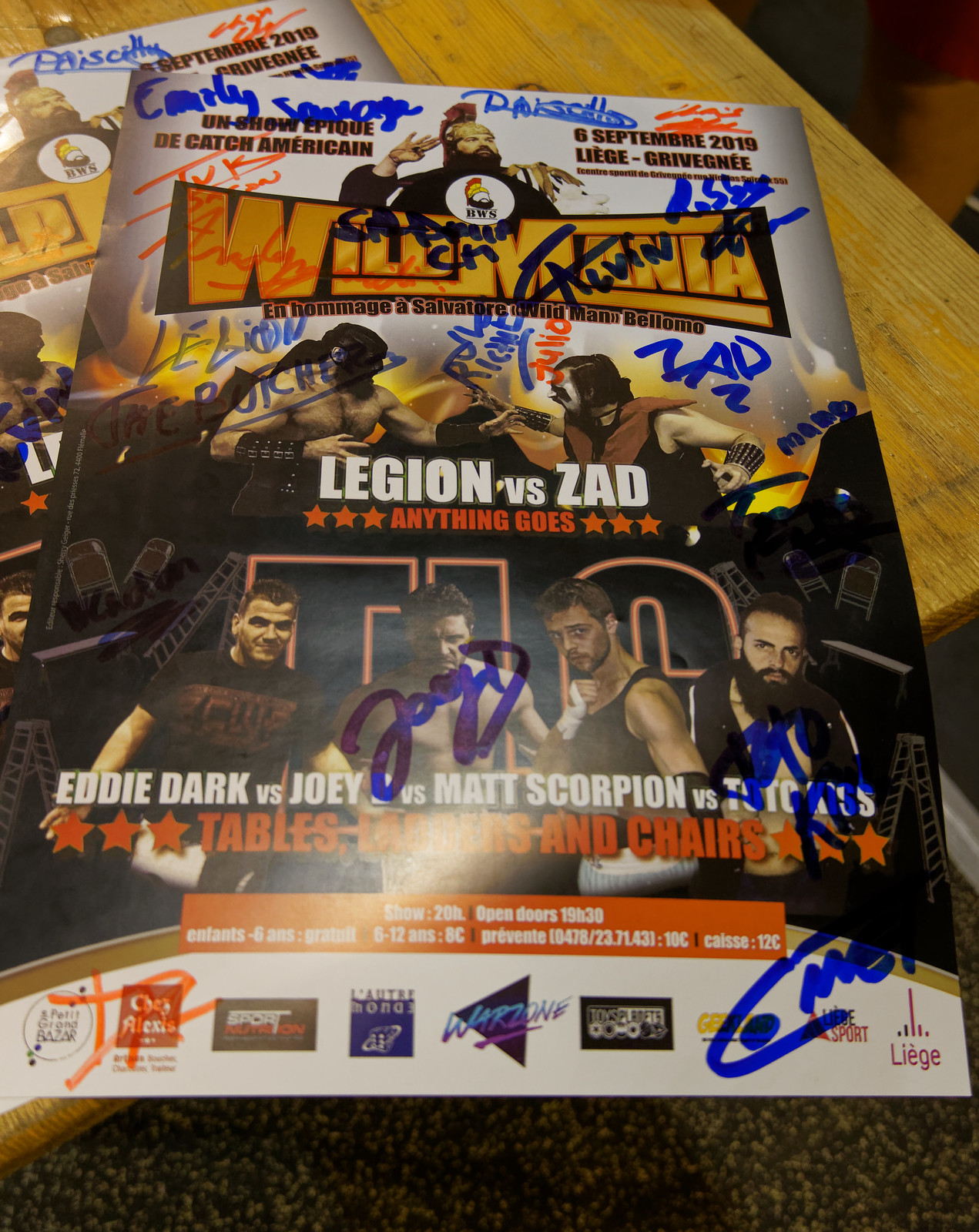The image depicts two autographed wrestling posters laid out on a light wooden tabletop, with a background of brown carpet and generic laminate flooring visible. The top part of each poster prominently displays the bold, blocky text "Wild Mania" in reddish-orange and yellow letters with black shadows. Below this title, two men are showcased in a confrontational stance: the left one, shirtless with black face paint and bracers, and the right one in black and red vest with clown-like face paint, both named "Legion" and "Zad" respectively. The phrase "Anything Goes" is emblazoned in red beneath them. The lower section of the posters features images of four tough-looking men poised for combat, their names listed as Eddie Dark, Joey, Matt Scorpion, and an unreadable final name due to a glare from an overhead lamp. The photos are autographed in blue and orange ink, adding a chaotic touch to the scene.